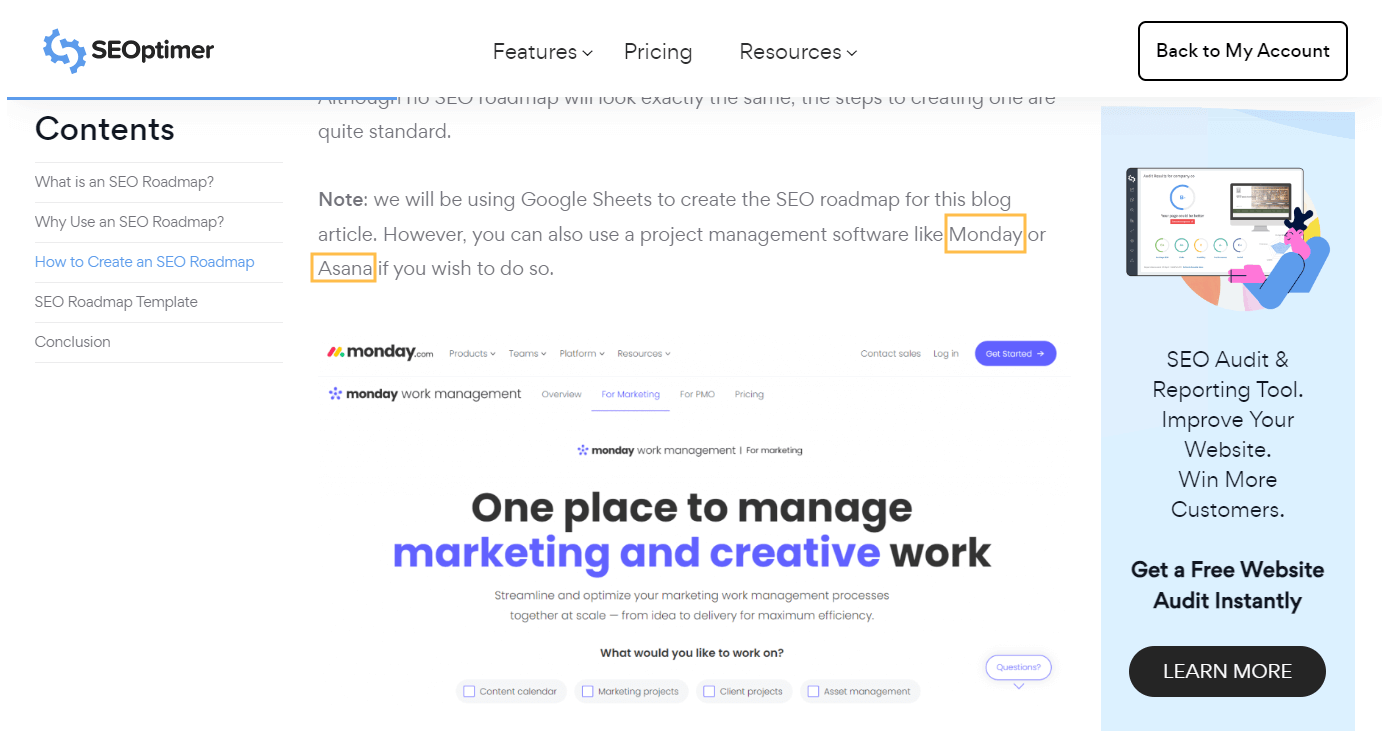**Caption:**

This computer screenshot features a predominantly white background with black and gray text. In the upper left corner, the text "SEO P Timer" is displayed, underlined in blue. Below this title, the section headings read: "Contents," "What is an SEO Road Map?" and "Why Use an SEO Road Map?". The clickable link, "How to Create an SEO Road Map," stands out in blue.

To the right, a note reads: "Note: We will be using Google Sheets to create the SEO Road Map for this blog article; however, you can also use project management software like Monday or Asana if you wish to do so." The words "Monday" and "Asana" are highlighted with a yellow triangle icon for emphasis.

Further down the page, in large bold letters, it states, "One place to manage marketing and creative work."

In the upper right corner, there's a black rectangle with the text "Back to My Account." Below it, a blue vertical rectangle displays an illustration of a person with pink skin and a blue body sitting in front of a screen. This section is labeled "SEO Audit and Reporting Tool: Improve Your Website, Win More Customers. Get a Free Website Audit Instantly." At the bottom of this section, a black button labeled "Learn More" is prominently displayed.